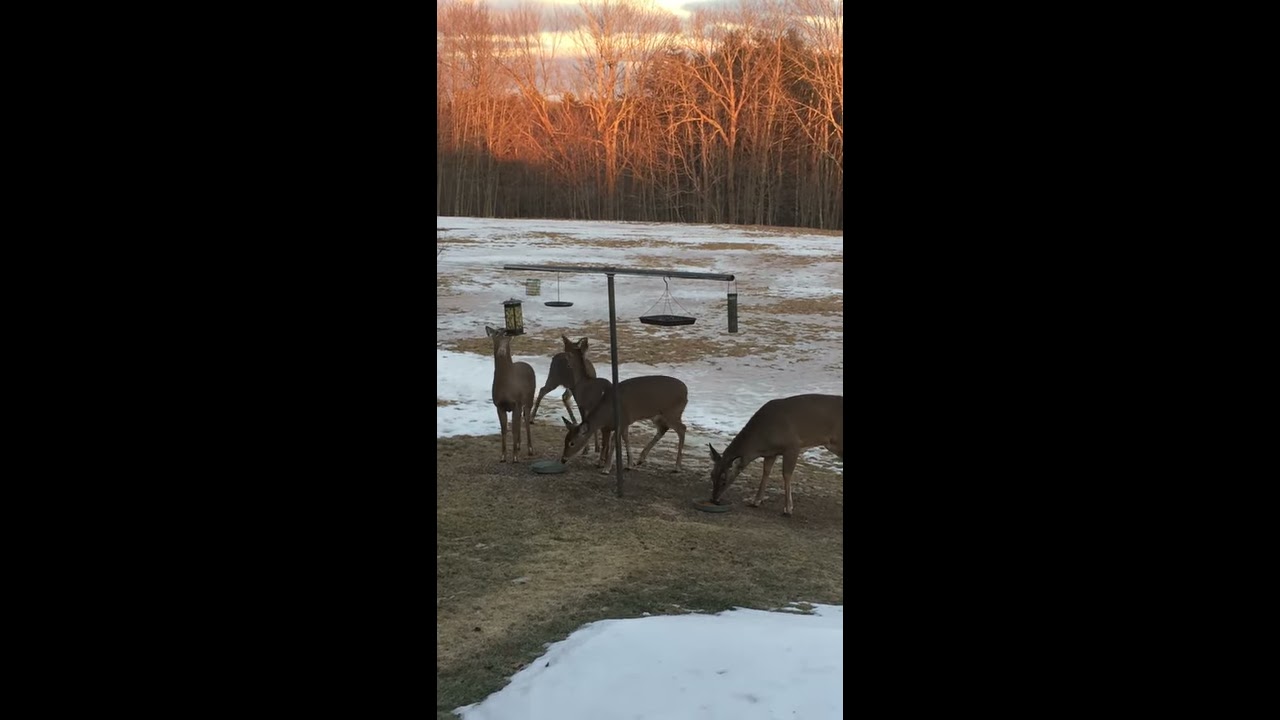A dawn landscape of a melting snow-covered field with patches of green and brown grass greets the viewer in this portrait-oriented color photograph. Central to the image are five medium-sized, hornless deer, gently feeding from a T-shaped deer feeder equipped with various metal pans. One deer looks straight at the camera, while the others are either eating or facing away. To the left of the feeder, there is also a bird feeder. In the background, a leafless forest stands in stark contrast to the dark, cloudy sky with the glow of the rising sun adding subtle illumination. This detailed and representational photograph is framed within a landscape-oriented black background, emphasizing the serene and realistic essence of an early morning in nature.